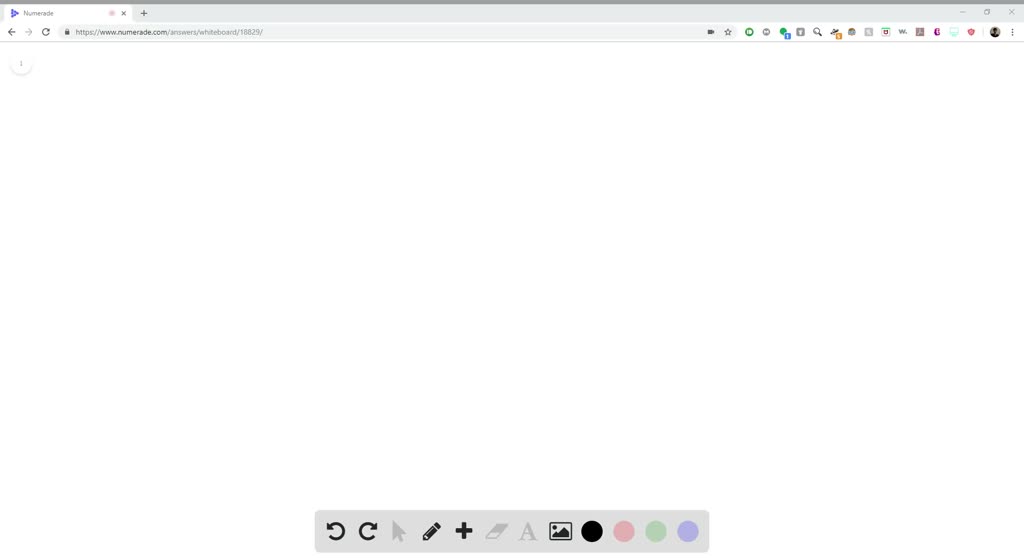The image is a screenshot of a website, specifically displaying a notepad section. At the top of the screen, a URL is shown but it is too small to be readable. The majority of the screen is filled by a blank, white notepad-like area, suggesting it is ready for user input. At the bottom of the screen, there is a toolbar that includes various interactive icons. These icons include a rewind and a fast-forward button, a mouse or clock symbol, a pen, and an eraser with a plus sign. Additionally, there are color options displayed in black, pink, green, and purple.